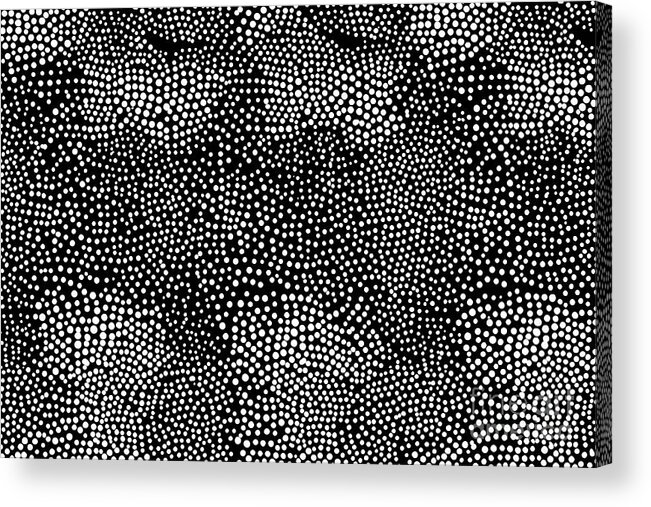The image depicts a piece of abstract artwork mounted on a canvas frame, displayed against a white background. The canvas itself features a striking design of countless small white polka dots scattered across a black background. These dots, varying in size and spacing, create a non-uniform pattern that gives an illusion of density variations. Some sections appear denser with white dots, while others allow more of the black canvas to peek through. The pattern continues around the edges, indicating that it is a wrapped canvas print. The artwork, lacking any identifying marks or signatures, possesses an optical illusion effect due to the overwhelming number of dots and their seemingly random placement. The piece is slightly tilted to the right, showcasing the black sides of the canvas, which adds to its unique and modern presentation, possibly suggesting it could be part of an art exhibit or for sale.